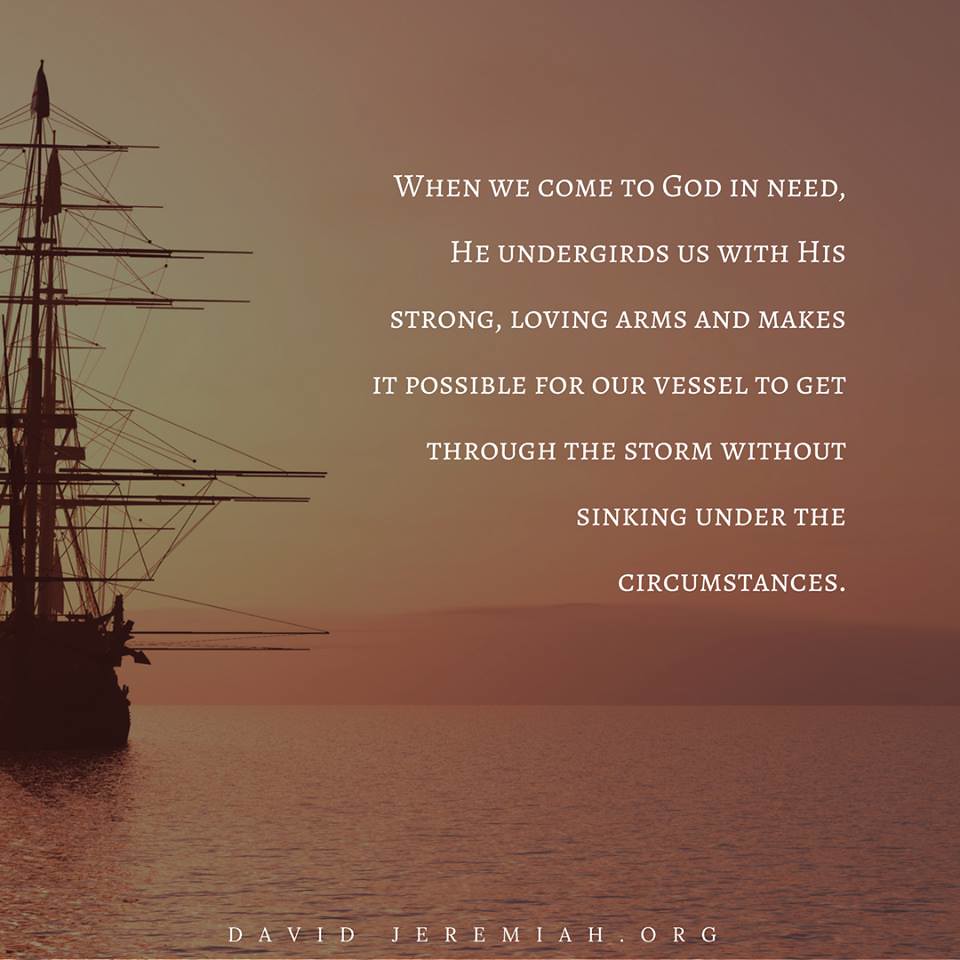This inspirational poster features a digitally generated image of a serene ocean scene set in muted, browns and yellowy tones, evocative of either an early morning sunrise or a late evening sunset. The focal point of the image is a large sailboat positioned on the left side of the frame, almost cut off, displaying tall masts. In the distant background, hazy waves or an indistinct mountain structure can be seen, enhancing the tranquil yet somber atmosphere. The sky and water both carry an orangish hue, reflecting the soft light conditions. The central theme of the poster is conveyed through white lettering that reads: "When we come to God in need, He undergirds us with His strong loving arms and makes it possible for our vessel to get through the storm without sinking under the circumstances." At the bottom center, the poster credits its source with "DavidJeremiah.org." Ideal for a contemplative space like a bathroom, this poster blends a calming visual with a comforting and powerful spiritual message.